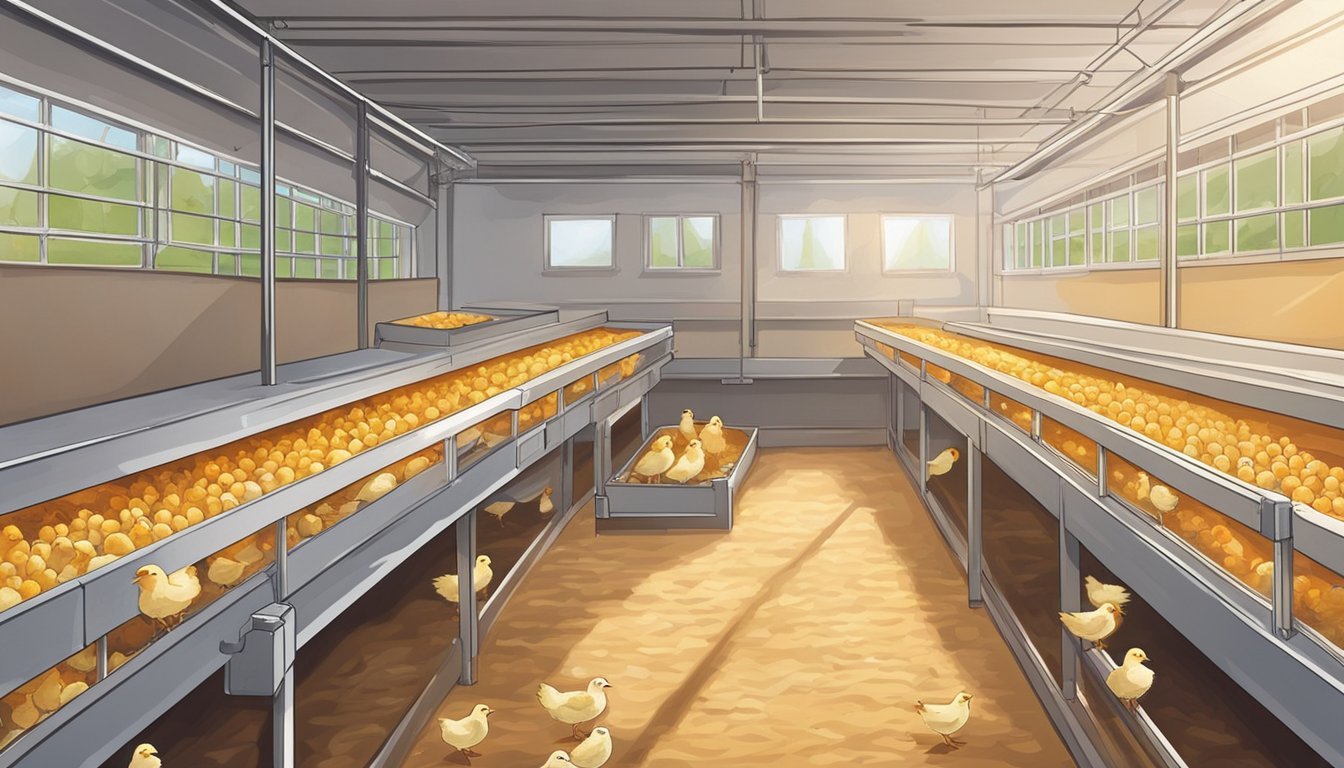The image depicts a busy hatchery inside a metal, rectangular building with a dirt floor. Hundreds of small yellow chicks are scattered throughout the space, both walking on the ground in the foreground and crawling in long trays on either side. The building features gray aluminum trays and overhead piping, suggesting a sturdy metal structure. Four windows at the end of the building, along with additional windows on the sides, allow bright sunlight to stream in, casting shadows on the dirt floor. Through the windows, greenery and bits of the sky are visible, indicating a spring or summer setting. In the background, a large container resembling a kitty litter box, possibly functioning as incubators, can be seen amid the plethora of chicks. The overall scene is slightly hazy from the intense sunlight shining through the windows.